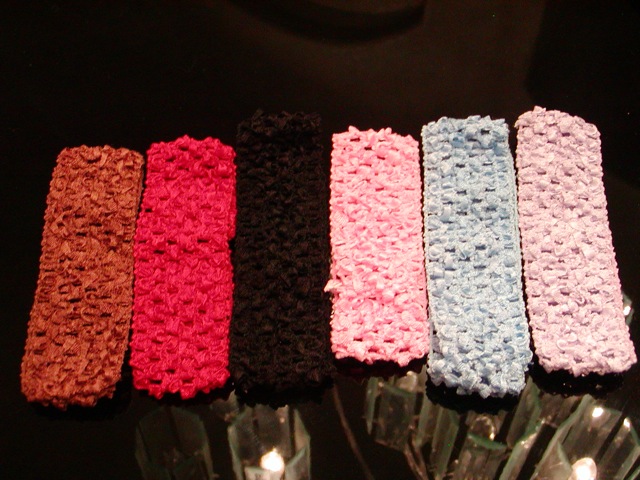A detailed photograph showcases six crochet headbands or bandanas meticulously aligned from left to right across the center of the image. Positioned against a dark brown or black background, these headbands exhibit a vibrant array of five distinct colors. Starting from the left, the first headband is a rust color, followed by red, then a black band that seamlessly blends into the background. Continuing towards the right, the sequence includes light pink, light gray-blue, and a very light gray-pink on the far end. Each headband is approximately 1.5 to 2 inches in width and about three inches in length.

Below the row of headbands, the scene is further adorned with small glass goblets, each containing large, white, Christmas light bulb-shaped ornaments. Most of these bulbs are turned off, maintaining a pristine white appearance, except for one in the center and one in the bottom right corner, which are turned on and emitting a warm, glowing light. The headbands rest atop a dark surface, possibly a table, which subtly reflects the ambient lights above, enhancing the overall indoor setting captured in a square-shaped photograph.